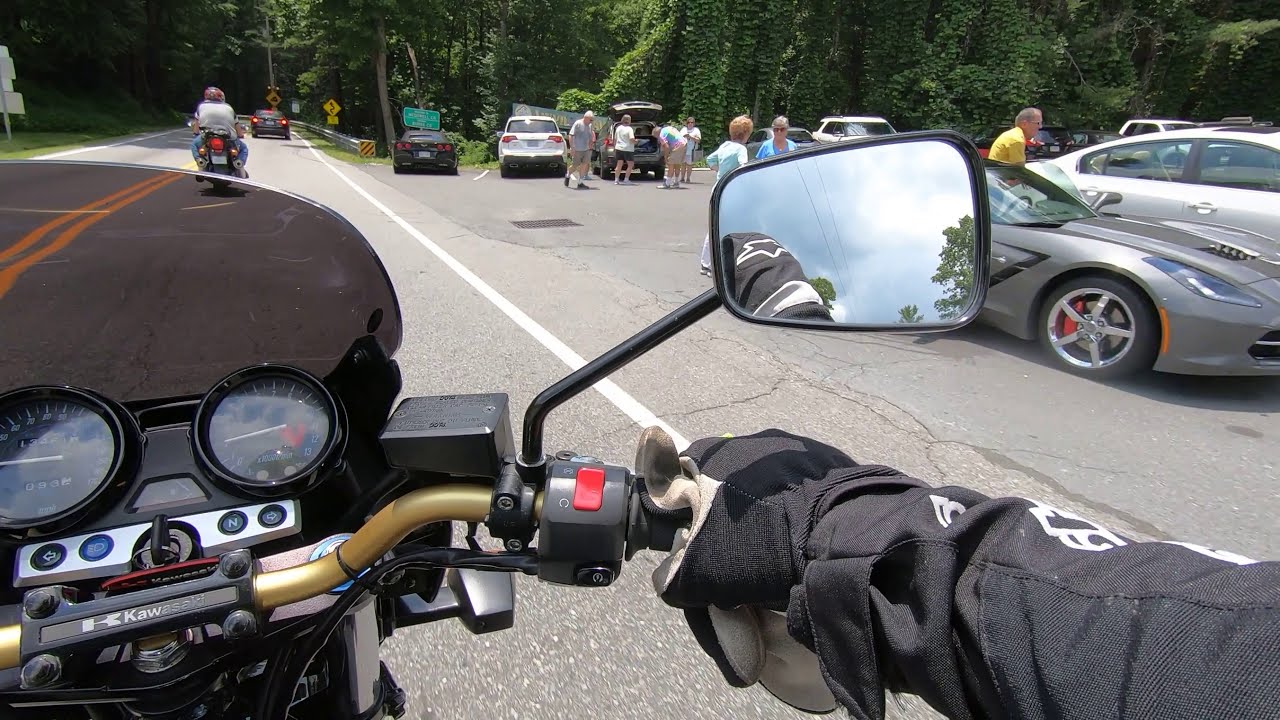The image captures a vivid, daytime scene from the perspective of a motorcyclist on a two-lane road. In the foreground, the motorcyclist's right arm, clad in a black long-sleeve jacket adorned with a white fox head emblem, grips the throttle. A black and white glove covers their hand. The golden handlebar and the dashboard, featuring a speedometer and other gauges, are also visible. A red switch is located to the left of the rider's glove. The rearview mirror, centered on the image, reflects a cloudy sky and part of the rider's shoulder.

In the midground, directly ahead of the rider, another motorcyclist and a car are seen moving in the same direction. To the left, near the double yellow lines that separate the lanes, the road extends forward. On the right side of the image, a parking lot is visible, packed with cars and people standing near their opened trunks, suggesting a scenic viewpoint or rest area. The surrounding scenery features a dense forest, framing the parking lot. The photograph, captured in the realistic style typical of a GoPro camera, offers a dynamic and immersive glimpse of a motorcycling journey through a picturesque area.